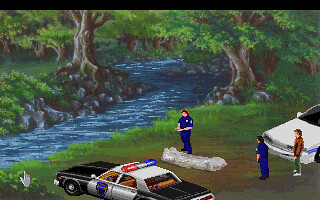This image appears to be a detailed, computer-generated scene from a video game. In the foreground, a black and white police car with red, white, and blue lights on its roof is prominently displayed. The car features a blue badge emblem on its white doors. Near the police car stands a short-sleeved police officer, hovering over what looks like a clear body bag. Another officer in blue is positioned nearby, off to the right. To their side, a person wearing a brown jacket, blue jeans, and white runners is observed standing beside a white car with a blue stripe down the side. 

The scene extends to a serene natural backdrop featuring a blue stream running through the middle. The stream is flanked by green grass and rocky outcrops at the water’s edge. Two large trees—rooted deeply into a rocky embankment—stand on either side of the stream, their green leaves extending skyward. The grass leads seamlessly up to the river bank, suggesting that the incident has drawn authorities to this tranquil yet ominous site, possibly to investigate a body found near or in the water.